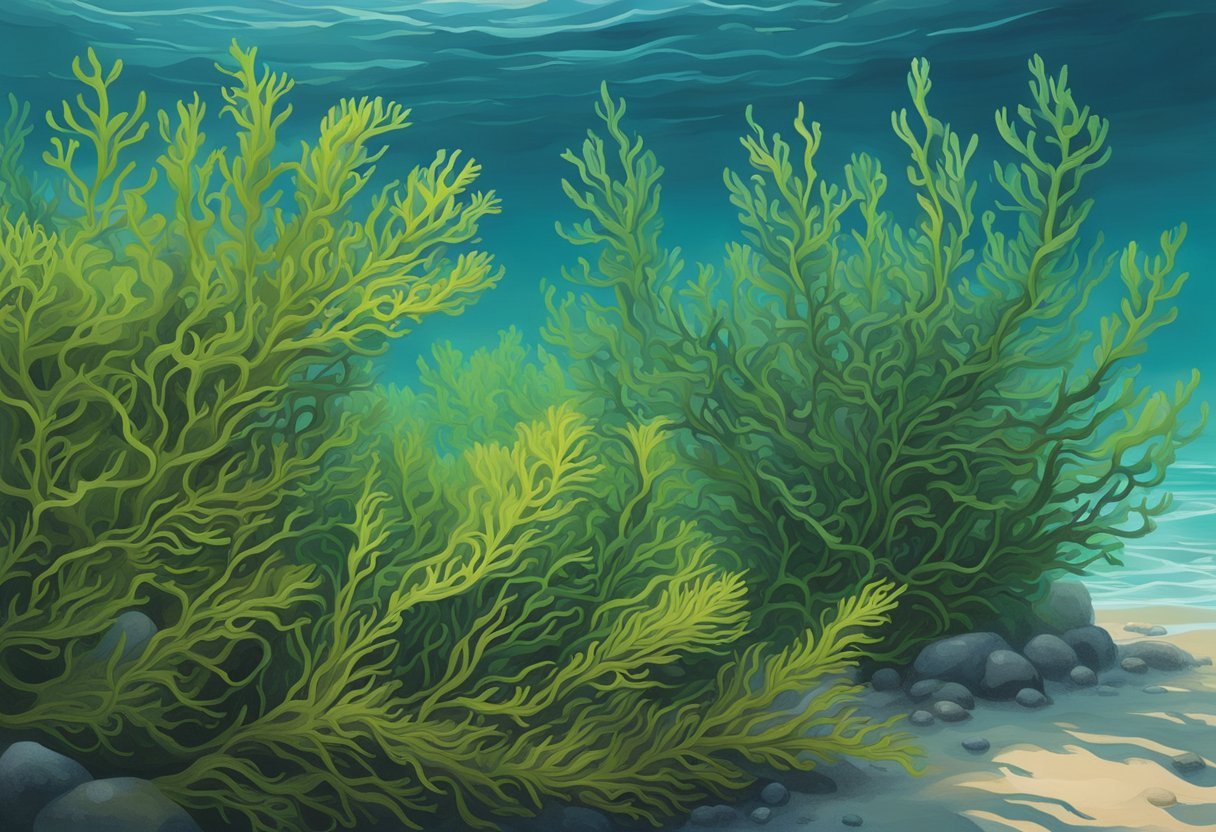The image is an illustration of an underwater view, capturing a tranquil scene of a tropical ocean floor. The water features various shades of blue, transitioning from a darker hue at the top to a lighter blue at the bottom, indicating different depths. The well-lit seafloor reveals a sandy bottom interspersed with an array of gray stones, varying in size, from smaller pebbles to larger rocks. These rocks are notably present in the lower right and left corners of the image.

Dominating the scene are numerous green, branch-like plants that resemble long, wavy noodles, spanning from the left side across to the middle, with a blank sandy section on the lower right. The plants on the left appear lighter green, while those on the right are slightly darker, their shadows casting intricate patterns on the sand below.

The painting, likely created with acrylics, intricately portrays the underwater environment, highlighting how light reflects and refracts, creating streaks of white and darker blue throughout the water. Numerous small, undulating waves with hints of white foam can be seen at the top, contributing to the serene and layered depth of this beautifully crafted seascape.